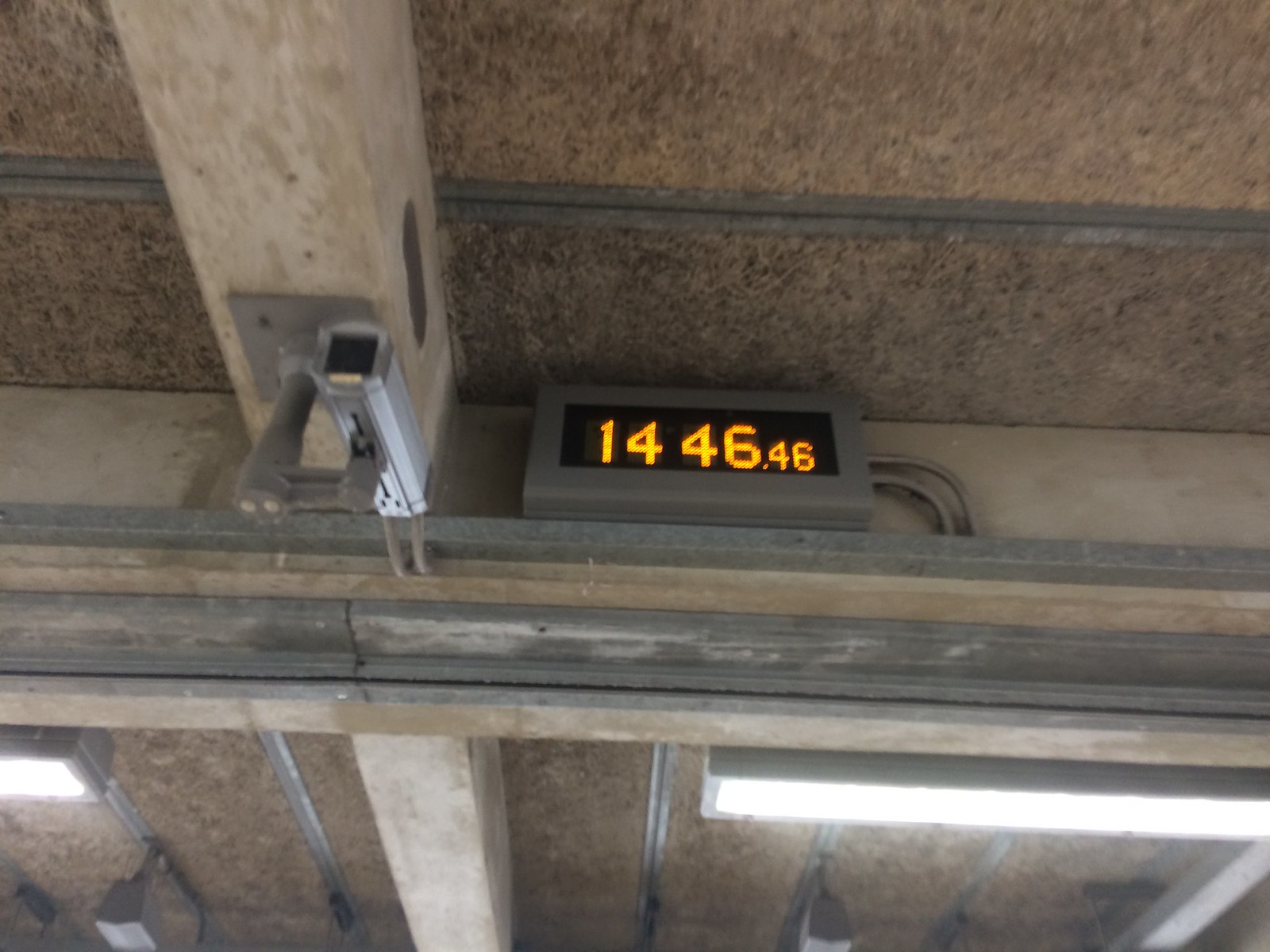The photograph captures the ceiling of what appears to be a parking garage, characterized by a grayish-brown cement texture. The ceiling features rough, holey surfaces and multiple cement support beams running both horizontally and vertically. Prominently displayed is a gray digital clock with bright orange numbers reading 1446:46, with a couple of cables extending from it into the ceiling framework. To the left of the clock, a small, silver surveillance camera with a cylindrical shape is mounted on one of the central cement beams. The environment is illuminated by long, thin, bright fluorescent lights typically found in office spaces or parking garages. The overall palette of the image consists of various shades of gray and light brown.